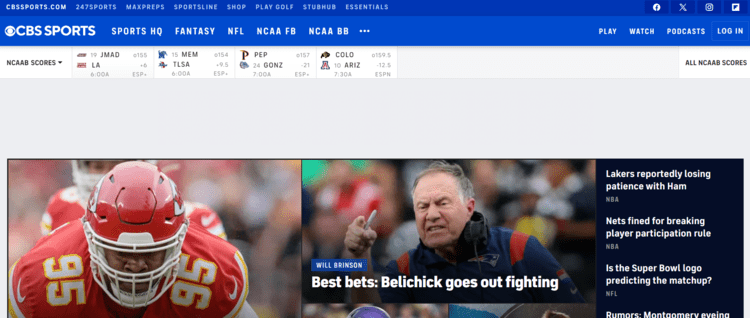This screenshot displays the interface of the CBS Sports website. At the top, there is a prominent royal blue navigation bar featuring the CBS Sports logo in white text. To the left of the text is the CBS logo, depicting an eye within a white circle. To the right of the logo are menu items labeled: Sports HQ, Fantasy, NFL, NCAA F8, and NCAA B8. Additionally, there are drop-down menus for Play, Watch, Podcasts, and Login.

Just below the navigation bar, a white ticker bar presents current scores for ongoing games, although the scores are too small to be legible. Beneath this, there's a gray, empty bar that serves as a divider.

The main content of the webpage is the front page of CBS Sports. Positioned on the left side of this section is an image of an African American football player in a red uniform and helmet, displaying the number 95 in white on his shoulders. To the right of this, there is a snapshot of an older Caucasian man, appearing visibly angry, making a pointing gesture. Below this image, white text reads: "Best Bets, Belichick goes out fightin'."